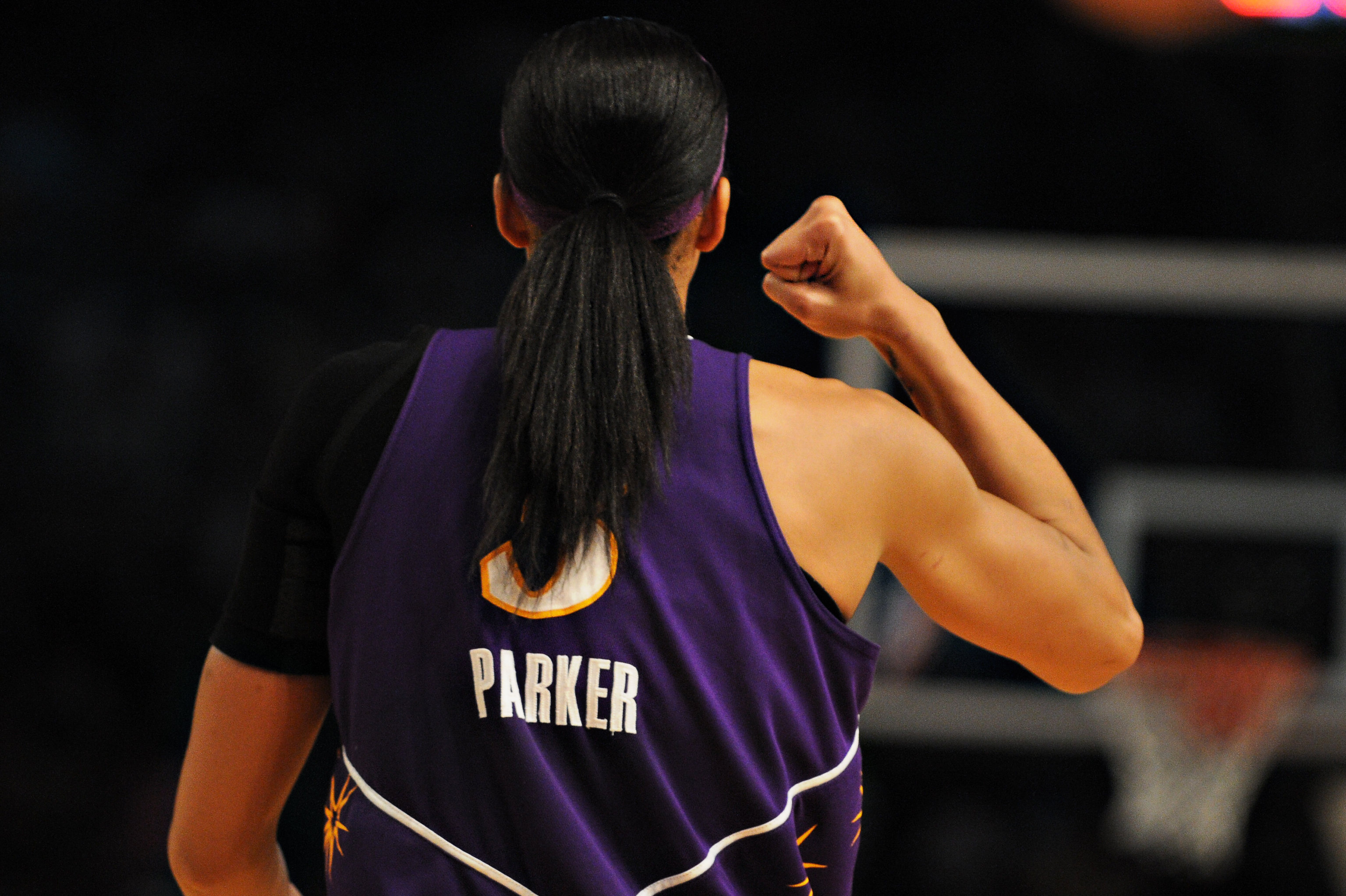The image captures the back view of a basketball player who appears to have just scored a goal. The player is clad in a navy blue jersey, which features white text that reads "Parker," along with the number "3" also in white but outlined in yellow. The player is identifiable by her long black hair and a purple headband. Her right arm is bent at the elbow with a fisted hand raised to elbow height, while her left hand is similarly positioned. A black arm strap is visible on her right arm. In the background, on the bottom right-hand corner, a basketball hoop is discernible against a dark backdrop.